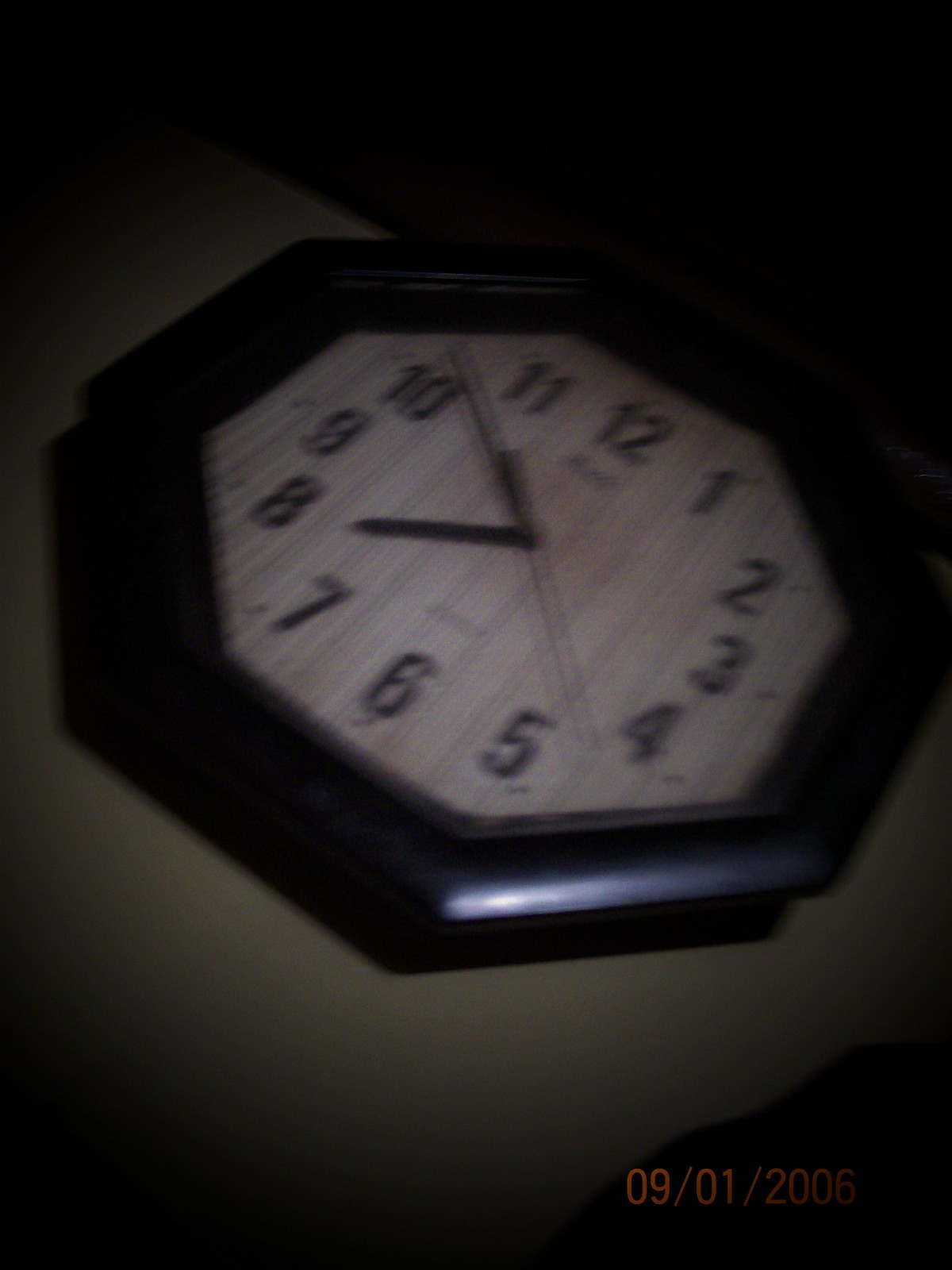This image is a dark and blurry photograph of an octagonal clock. The clock, which appears to be mounted on a wall that might be greenish in color, features a thick black border enclosing a faded, possibly dirty, white face. The interior of the clock resembles a fence due to vertical stripe patterns running from 12 o'clock to 6 o'clock. The clock displays black numbers, ranging from 1 to 12, and shows the time as approximately 10:39, with the hour hand between 10 and 11, the minute hand near 8, and the second hand positioned around 52 seconds. There is a faint, potentially superimposed, date in the bottom right corner in an orange or dark red font, indicating 09-01-2006, though the last numeral is somewhat faded and unclear. Despite the image's poor lighting, the clock’s details are distinguishable while the background remains shrouded in darkness.